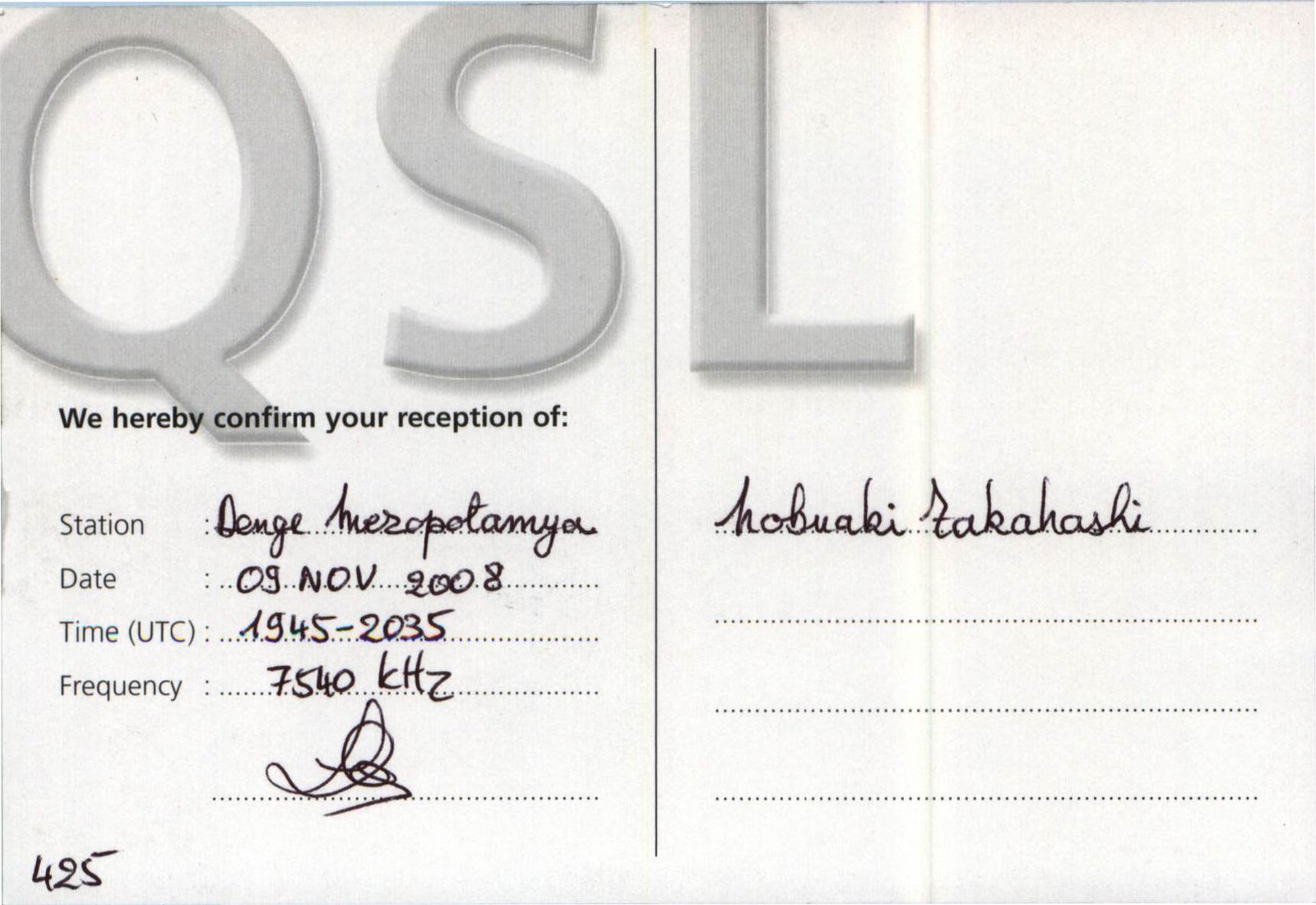This image features the backside of a wide, rectangular postcard with a slightly off-white background that becomes pinkish towards the top, especially on the top right side. A prominent crease runs slightly to the right of the center of the card, appearing grayish-yellow. At the top left, partially cut-off, are three large, gray, 3D-looking letters that read "QSL". 

The postcard is divided into two halves by a vertical line. On the left half, a bold black font reads, "We hereby confirm your reception of," followed by several lines filled in with black pen. These lines detail the station as "Dengue Aeropotamia", the date as "05 November 2008", the time as "1945 to 2035 UTC", and the frequency as "7540 KHZ". 

On the right side of the postcard, there is a name written as "Hobuaki Takahashi". Additionally, the number "425" and an initial signature are mentioned towards the bottom, all scripted in black.